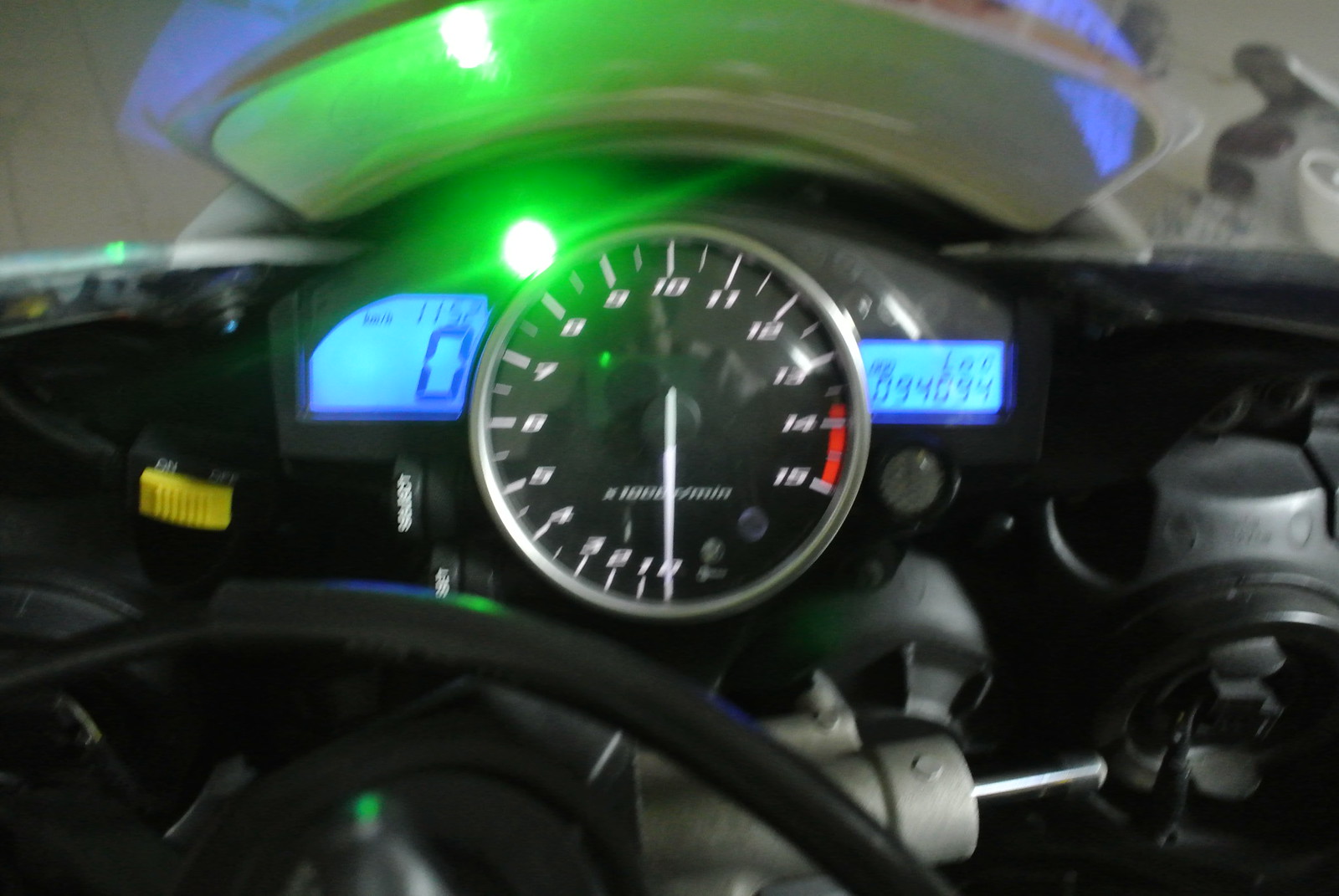This macro photograph showcases a close-up of a vehicle's dashboard. The image captures the intricate details of various components, though it does not reveal the dashboard in its entirety. At the top of the composition, there is a curved piece, seemingly white, but illuminated by an underlying green light, casting a green hue across the surface.

Beneath this, there is a round gauge, slightly out of focus. The gauge features numbers starting from zero and increasing in single increments up to 15. Although the label on the gauge is indistinct, the white indicator line points to zero, suggesting that the engine is currently off. Adjacent to the 14 and 15 marks lies a red zone, likely signifying a cautionary range where operating there might necessitate slowing down.

To the right of the round gauge, a blue-lit screen displays numerical data. Similarly, another blue screen to the left shows a solitary zero. 

Below these digital readouts, the image provides a glimpse under the hood, revealing various engine components. The engine area is populated with black hoses, possibly belts, and other silver or gray mechanical parts. A notable detail is a yellow slider-like component, whose specific function remains unclear.